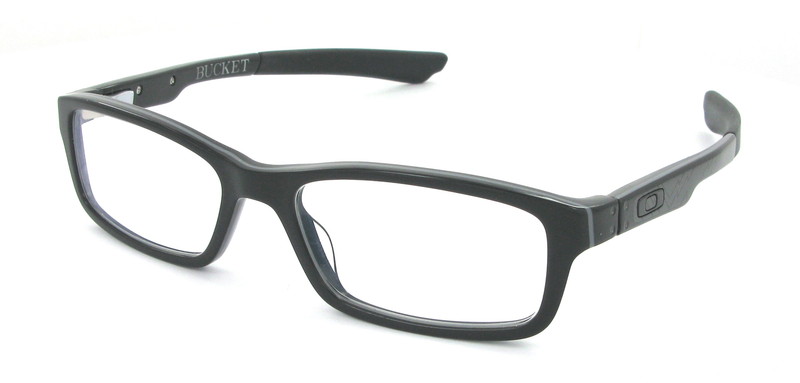This color photograph, in landscape orientation, features a pair of angular, slightly curved, black eyeglasses prominently displayed against a pristine white background, creating a stark and clean visual. The glasses exhibit a realistic, representational photographic style, typical of professional product photography. The thick, black plastic frames are rectangular in shape, extending into black plastic arms that curve inward toward the ears. The frame appears to be designed for men and is angled from the top left to the bottom right. 

Distinctively, on the inner portion of the right arm, the brand name "Bucket" is clearly inscribed in white text. Near the brand name, there are two visible small screws, adding to the structural details of the glasses. Additionally, the right side of the frame features a small rectangle adjacent to another rectangle. The nose piece is simplistic and flat, without any additional padding or design elements. While the glasses appear sharp and clear, there is a subtle and unusual aspect to the glass itself that hints at a unique or specific design feature, though it's not immediately apparent. 

Overall, the minimalist approach of the white background serves to enhance the detailed and meticulous depiction of the eyeglasses, making them the absolute focal point of the image.